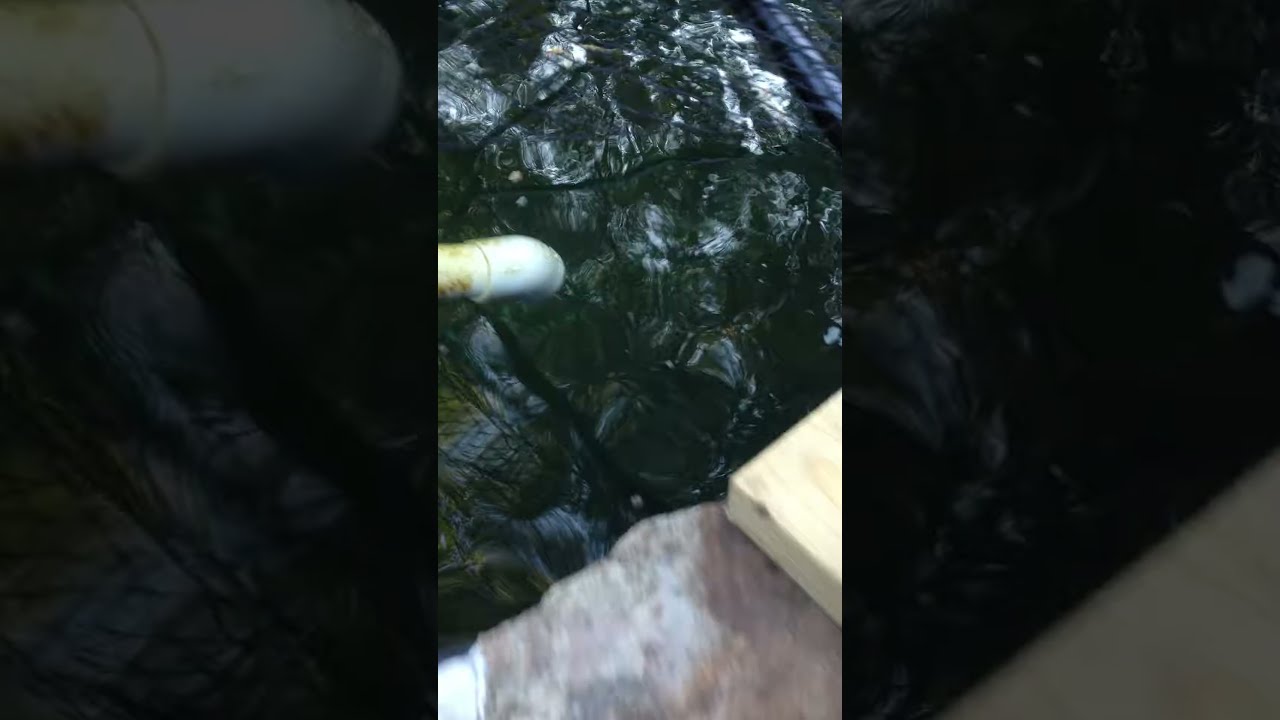The image is a slightly blurred close-up of a black and shiny object that resembles coal, possibly a fossilized foot, with a tortoise shell-like texture. An index finger, sporting a surgical glove, is seen pointing at or touching the object. Surrounding this central image, there are two vertical panels, each occupying about a third of the photo's width, displaying blown-up and darkly underexposed close-ups of the object's sides. On the right side, the black structure that might be a stone or tar-like substance appears to extend into the frame, suggesting a diagonal flow, possibly splashing into turbulent water beneath. The background includes elements like a red stone surface and a light-colored maple board, completing the detailed and multi-perspective view of the scene.